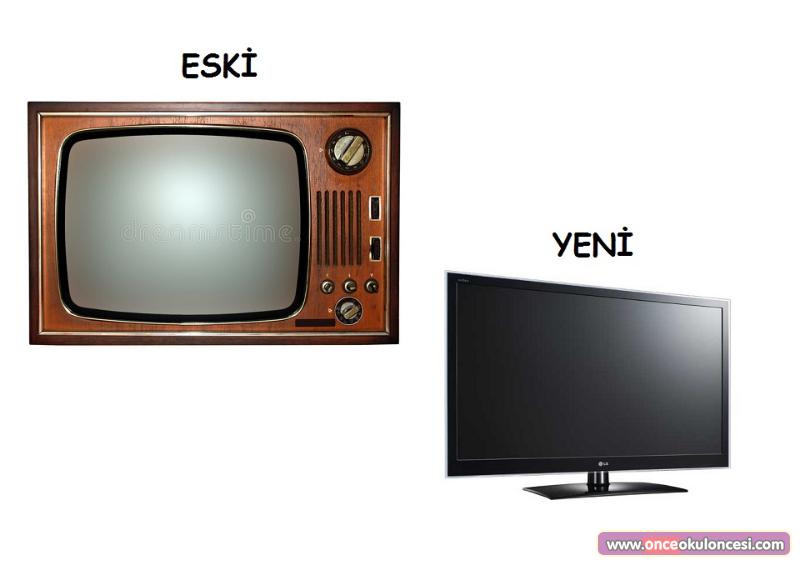This image features two distinct monitors placed against a solid white background. In the top left corner, there's a vintage television characterized by wood grain paneling, chrome knobs, a speaker, and buttons, evoking a sense of several decades past. Above this vintage TV is the word "ESKY" in all capital letters, written in Comic Sans font. 

In the bottom right corner is a modern flat-panel desktop monitor with thick bezels, positioned at an angle. The monitor, in all black with a small flat stand, has the word "YENNY" (a possible misspelling or variation of "YENI") written above it in a bold script font with an umlaut over the "i". Below this modern monitor and to its right is a URL displayed in a colorful rectangular box, variably described as lavender or red, reading "www.onceokolensky.com."

The image juxtaposes technology from different eras, set against a minimalist background, possibly indicative of a hobbyist's collection or an online showcase. The colors observed in the image include white, black, brown, tan, gray, pink, and purple.